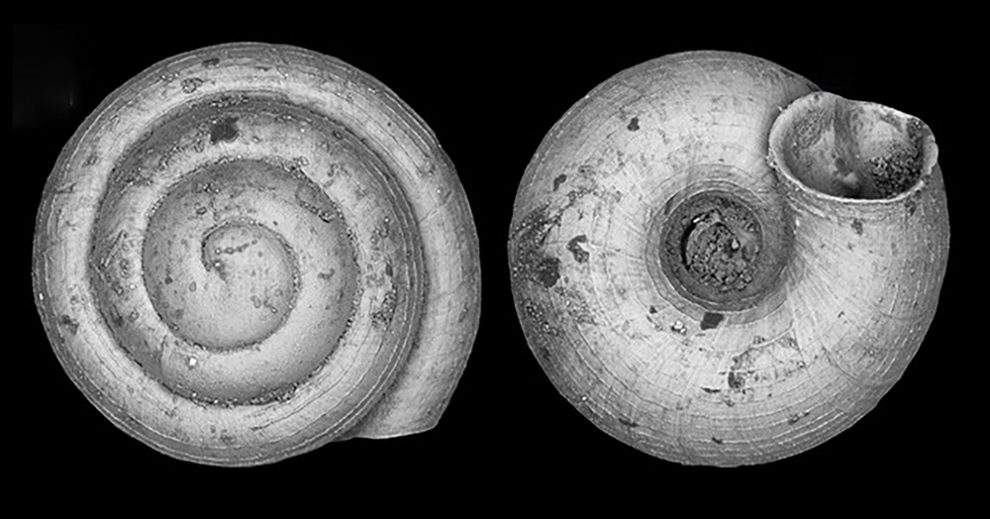The photographic black-and-white image features a highly detailed close-up of two nautilus shells against a dark grey background. On the left side, the shell is oriented to display its top surface, revealing a central swirl that spirals outward in a counterclockwise direction, complete with numerous pits, markings, and gouges suggestive of natural wear and debris. On the right side, the shell is shown from its bottom perspective, highlighting the cylindrical opening through which the creature would emerge, and similarly exhibits numerous cracks, discoloration, and rough textures. The image appears to be magnified, offering clear visibility of the intricate details and textures of both the front and backside of the nautilus shells. There is no text present in the image.